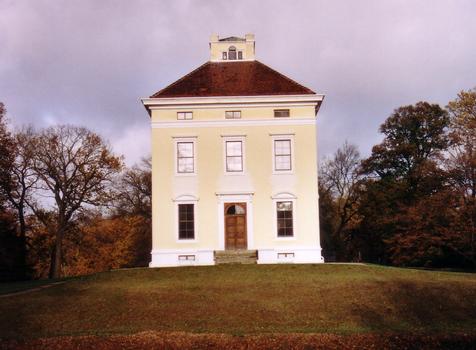This is an image of a small, cream-colored house perched atop a hill, framed by a forest with both leafless hardwoods and evergreens under a cloudy, gray sky. The house is a mix of Victorian and Federalist styles, featuring two full stories with an attic, making it effectively a three-story structure. The facade has a brown front door, reached by a set of stairs. The first floor has two large dark windows with white decorative tops, while the second floor has three windows with white shades. Just beneath the dark brown roofline, there are small half transom windows leading to what appears to be an attic or a lookout room. The structure is blocky and made of what looks like cement with white gutters. There is a hint of sunlight or some form of light illuminating the front of the house, giving it a slightly ethereal glow amidst the somber, cloudy backdrop.